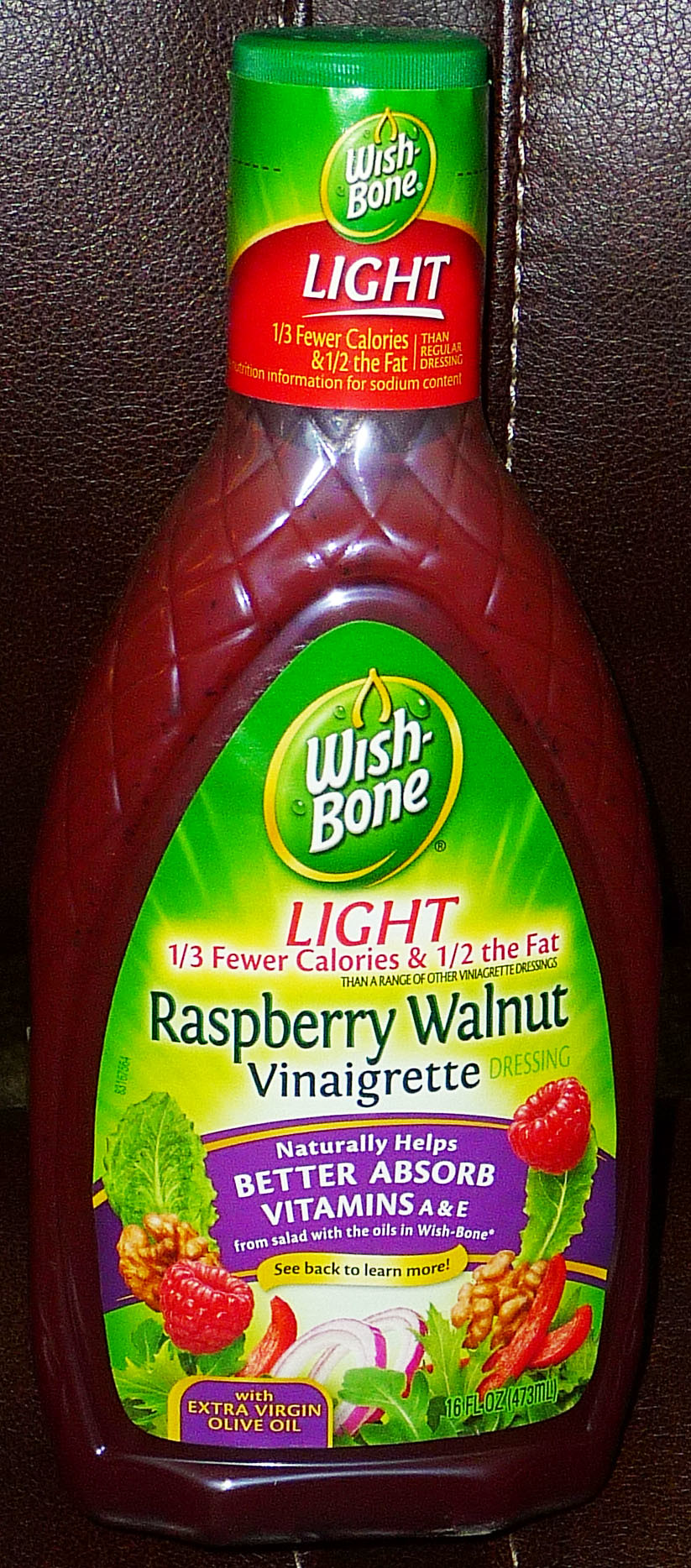The image showcases a bottle of Wishbone brand Raspberry Walnut Vinaigrette, comfortably positioned on the back corner of a leather couch. The amber-hued leather upholstery serves as a muted yet luxurious backdrop that contrasts beautifully with the vibrant vinaigrette. The bottle itself features the recognizable Wishbone logo emblazoned near the top, complete with their signature green wraparound design. Below, a larger, central label boasts details about the product: it highlights the "light" formula with one-third fewer calories, augmented with extra virgin olive oil. The vinaigrette takes on a rich, red tint, suggestive of its raspberry essence, visually complemented by images of fresh raspberries on the label. Additional text indicates the vinaigrette's health benefits, specifically its ability to naturally help absorb vitamins A and E better.